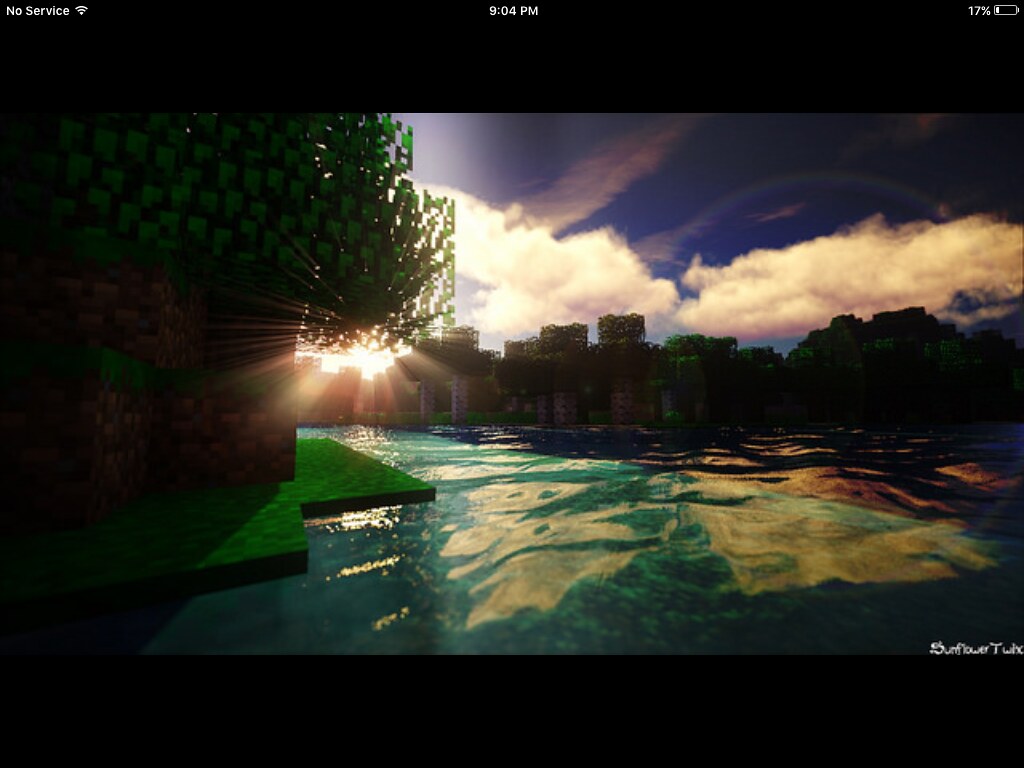A screenshot from a smartphone displaying a scene from a game is showcased amidst a black background. The top of the screen indicates "No Service" on the left, a time of "9:04 PM" in the center, and a battery level of 17% on the right. The central image depicts a vibrant, pixelated landscape reminiscent of Minecraft, featuring green land, block-like trees, and cliff sides contrasted against realistic-looking water and sky. At the bottom right corner, partial text reading "Sunflower" followed by a cut-off "T" suggests the name of the game or a related element.